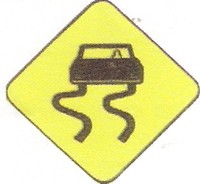This image features a prominently displayed road sign with a diamond shape, resembling a square turned on its point. The sign is outlined in a subdued black color, creating a clear but not overly bold contrast against the background. The interior of the sign is filled with a vibrant, sunny yellow hue.

At the center of the yellow backdrop, there is a simple sketch-like illustration of a car. The car's hood and main body are depicted with elementary shapes—a rounded front and a boxy outline for the main structure. A small arch at the front of the car indicates the presence of a driver.

From the front tires of the sketched car, two squiggly lines extend outward, symbolizing a winding or slippery road ahead. The background of the image is a blank, white computer screen, further emphasizing the bright and cautionary nature of the sign.